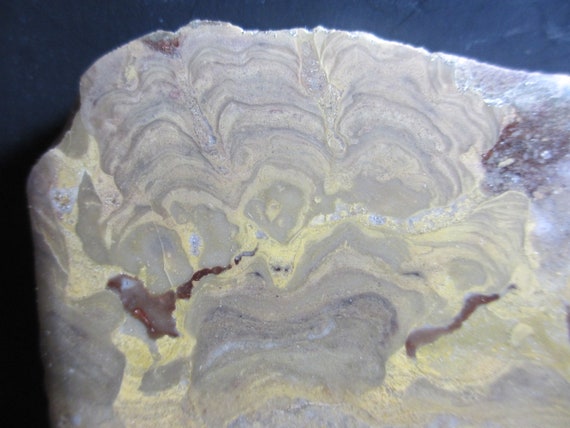This image captures a highly detailed close-up of a polished stone with a distinct and visually appealing appearance. The stone, possibly used for a tabletop, displays a unique grain pattern reminiscent of wood. Its smooth, flat surface contrasts with the jagged, chipped edges towards the top. The stone's composition includes a harmonious blend of wavy lines and layers in various shades of gray, cream yellow, and white, suggesting an intricate, flowing texture. Additionally, maroon, rust, and vibrant burgundy hues intermingle with occasional dark and light purples, adding depth and richness. The background, predominantly blue and light blue, fades to black in the lower left, highlighting the stone's complex, organic patterns.